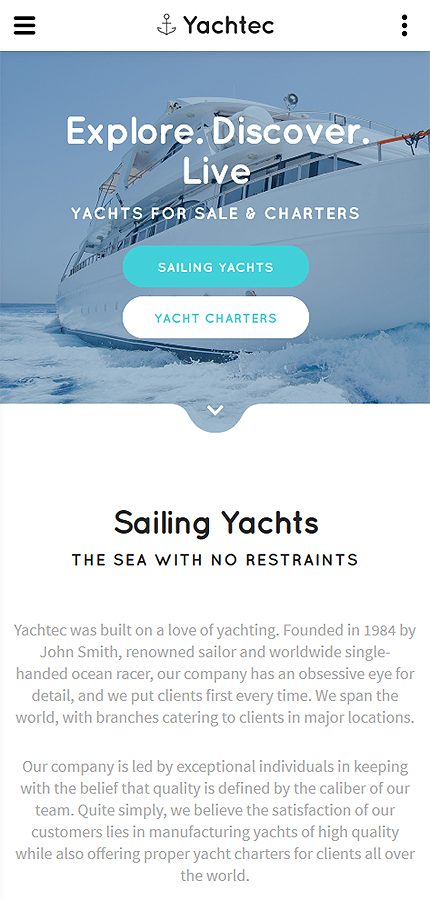At the top of the page, there's a white header with three horizontal bars for navigation options. Adjacent to the left is a gray anchor icon labeled Yacht Tech. On the top right-hand corner, there are three clickable bubbles. The main image features a light blue-tinted visual of a large, white yacht slicing through the water, creating a dynamic blend of white and blue waves. A hint of red is visible on one of the railings on the side, while plentiful glass elements reflect the surrounding environment. The yacht appears to be two stories high.

Centrally positioned on the yacht image are the words "Explore, Discover, Live, Yachts for Sale, and Charters," accompanied by two clickable links titled "Selling Yachts" and "Yacht Charters." Below this, a dropdown menu is presented. The page's content continues with a white section featuring black text that reads, "Selling Yachts to Sea with No Restraints." Complementing this is a gray-text passage that details Yacht Tech's history and philosophy. 

"Yacht Tech was built on the love of yachting, founded in 1984 by John Smith, renowned sailor and worldwide single-handed ocean racer. Our company has an obsessive eye for detail. We put clients first every time. We span the world with branches catering to clients in major locations. Our company is led by exceptional individuals in keeping with the belief that quality is defined by the caliber of our team. Quite simply, we believe the satisfaction of our customers lies in manufacturing yachts of high quality while also offering proper yacht charters to clients all over the world."